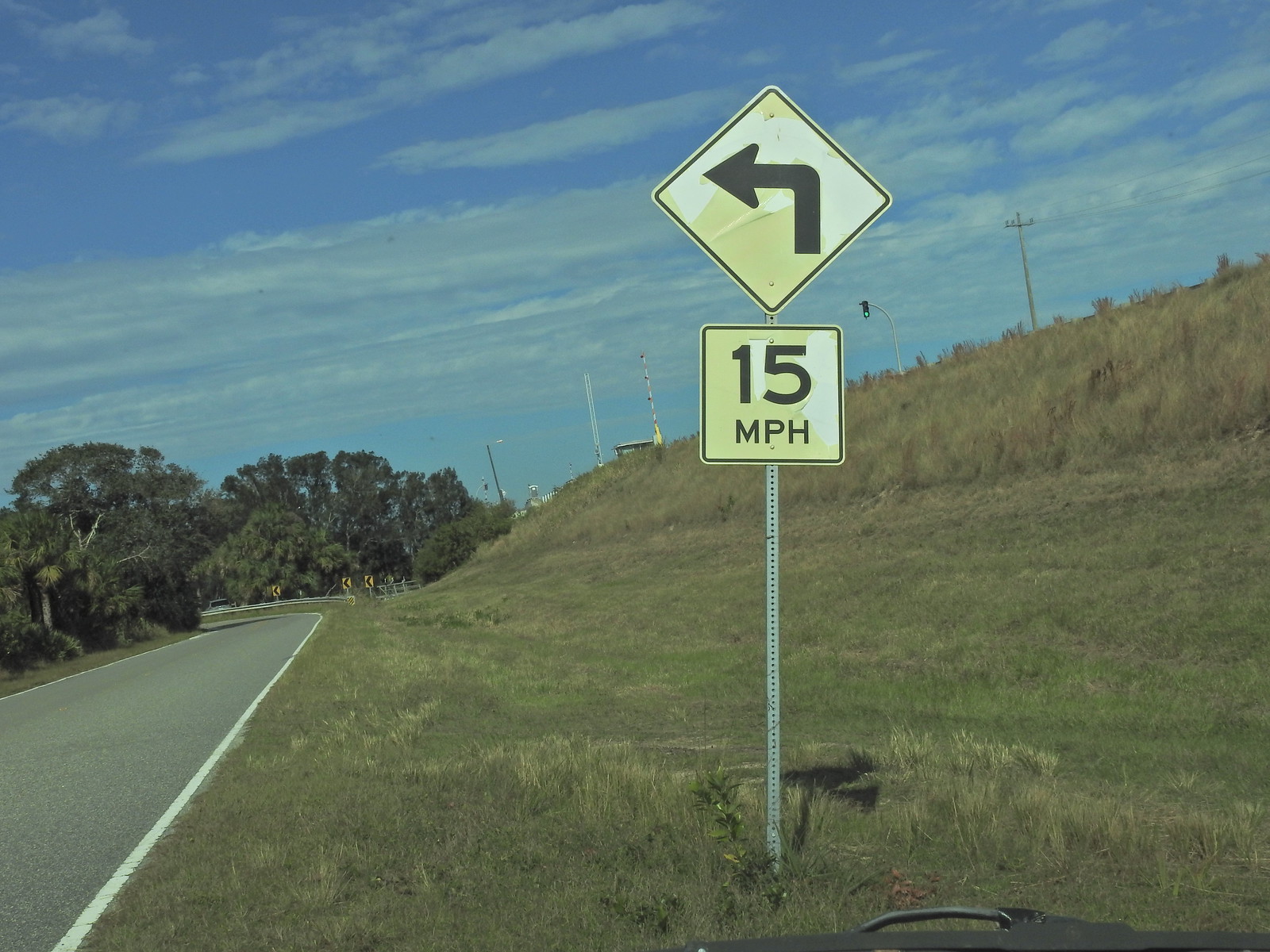This detailed photograph captures a single-lane roadway winding into a lush, tree-filled distance. The road, marked by a solid white line on its right, curves gently ahead, disappearing into verdant greenery. To the right of the roadway, a grassy hill rises, adding to the serene, natural ambiance of the scene. Mounted on a metal pole by the roadside, a conspicuous yellow diamond-shaped traffic sign with a black arrow indicates a left turn. Directly beneath this, a square yellow sign with black text limits the speed to 15 MPH. The entire scene is bathed in a subtle haze, with a clear blue sky overhead adorned by streaks of white clouds, enhancing the photograph's tranquil outdoor setting.